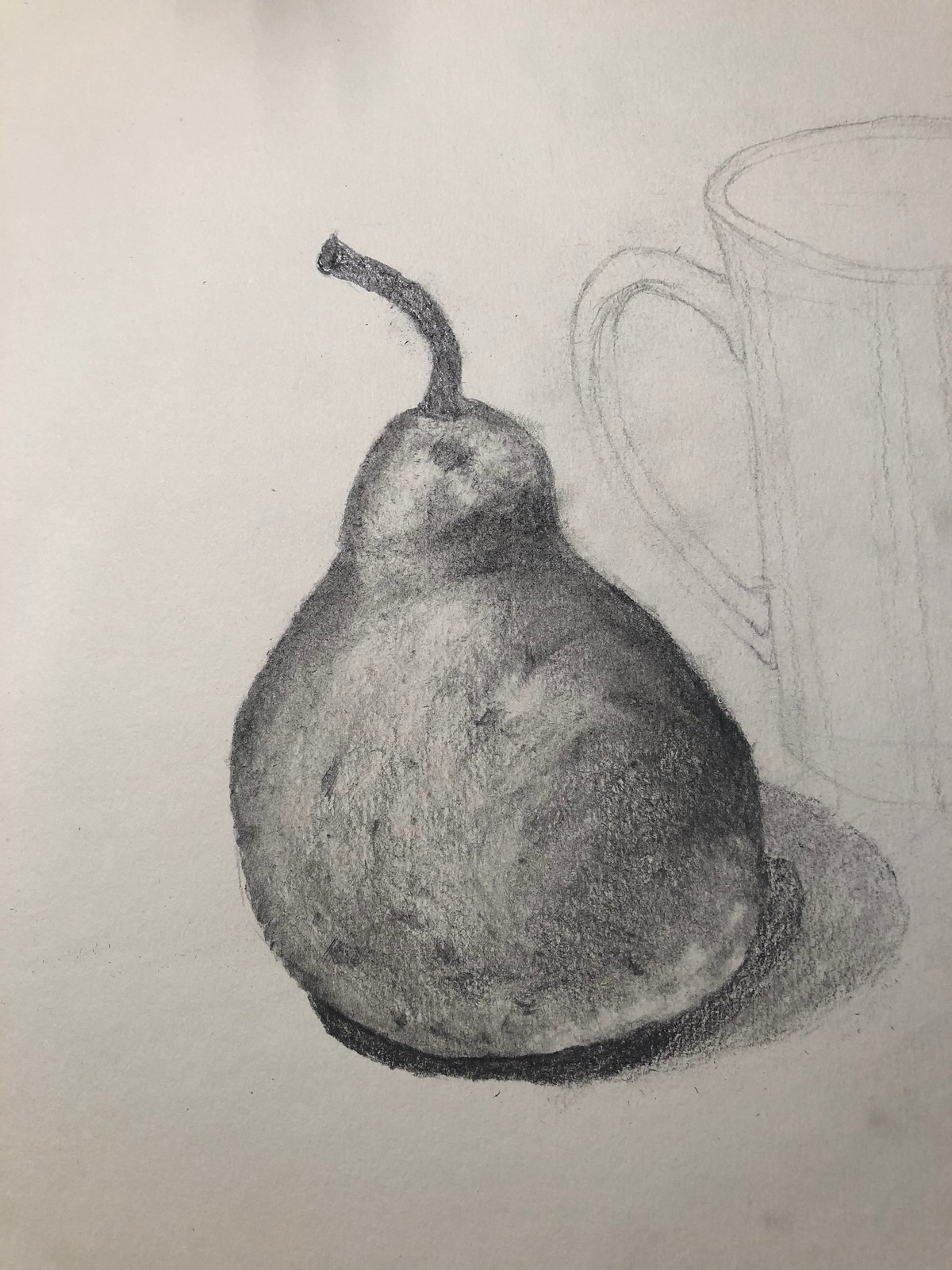This hand-drawn artwork, created with pencil and possibly some charcoal, showcases an intriguing still life composition set against a light gray background with some hand smudges. The central focus of the piece is a prominently detailed pear that features a heavily shaded, bulbous bottom narrowing towards the top, with a long, slightly bent stem extending out to the left. The pear rests on a well-defined shadow or perhaps a black base, adding depth to the drawing. To the pear's right and slightly above, there is an outline of a distinctive handled mug. The mug, taller than the pear, has an irregular, asymmetrical top and a noticeably curved handle that is sketchily rendered, giving it a unique, less defined appearance compared to the pear. Adjacent to the mug is a beaker, also sketched with light lines, providing a balanced contrast between the understated and the vividly detailed elements in this captivating pencil sketch.